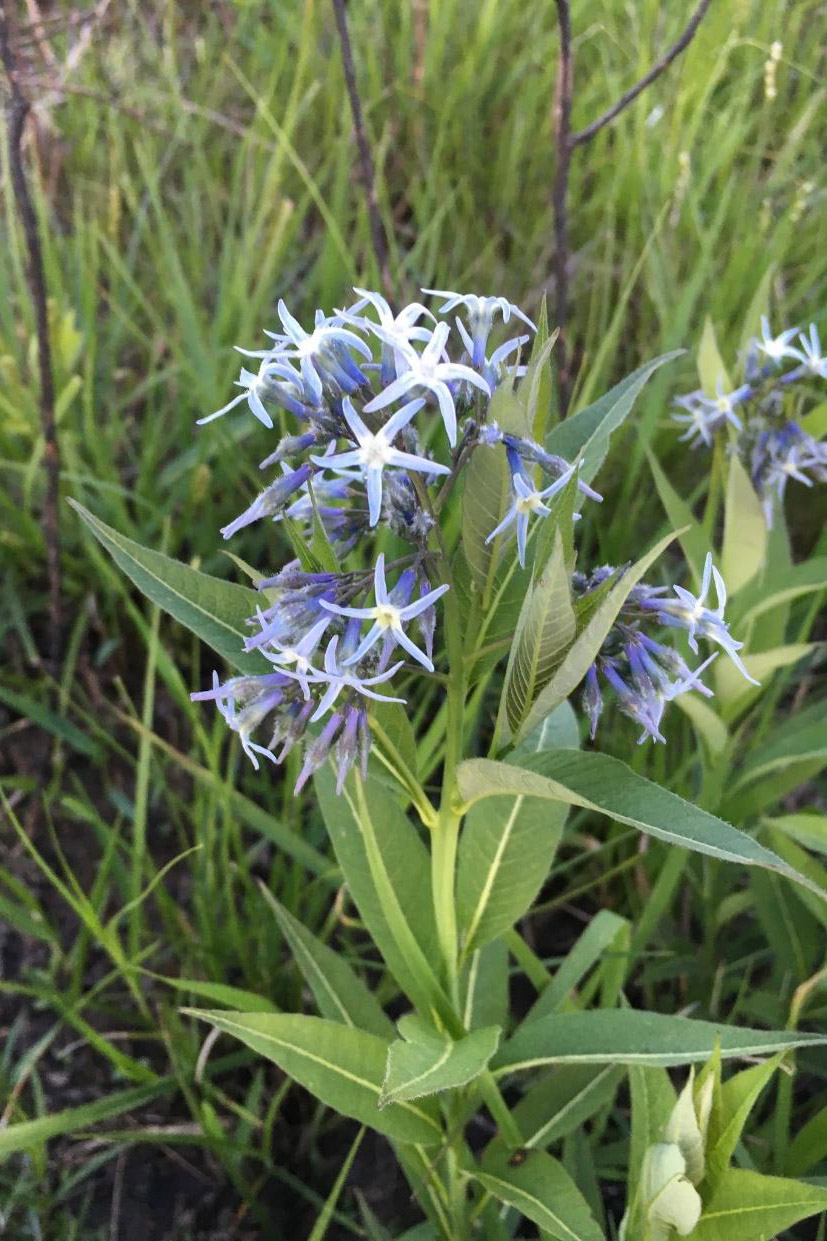This close-up photograph, taken outdoors during the daytime, features a vibrant blue star flower plant growing amidst a thick carpet of green grass. The plant, with its tall green stalk tinged with yellow undertones, rises centrally through the frame, reaching about three-quarters of the way up. Surrounding the stalk are long, thin elliptical leaves, dark green on top with prominent yellow veins and lighter green underneath. At the top of the stalk, clusters of starfish-shaped flowers with five pointed petals display a stunning gradient of purple, blue, and white, with yellowish-white centers. Some flowers appear fresh and vibrant, while others show signs of wilting. The background is a blur of green, accented with the occasional yellow grass blade and scattered dead twigs, indicating a sunny day with highlights reflecting on the foliage.